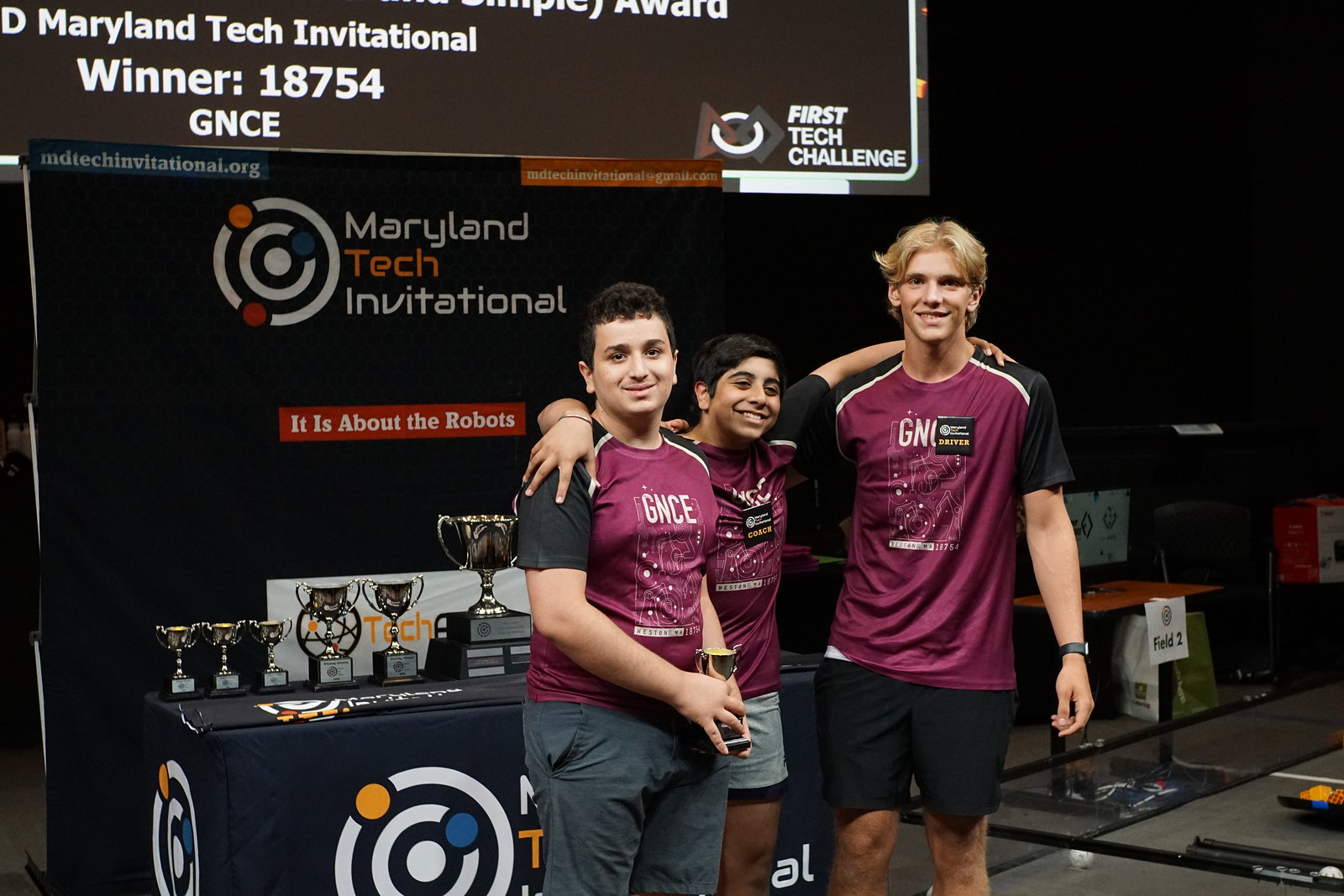In this vibrant photograph, three teenagers—two white and one South Asian—stand proudly, dressed in matching maroon and black t-shirts emblazoned with "GNCE." They are likely celebrating a victory at the "Maryland Tech Invitational," as indicated by the sign behind them. The sign above them, reading "First Tech Challenge," suggests a robotics competition. Their joyful expressions and embraces further imply a triumphant moment, with the teen on the left holding a trophy. The guy in the middle, who is shorter, has his arms around his friends, signaling camaraderie. Behind them on a blue shelf are multiple trophies, reinforcing the competition's atmosphere. The black poster behind them features a striking logo with orange, red, and blue concentric circles and the phrase "It's all about the robots" beneath a red-background rectangle. Additionally, their shirts feature roles such as "driver" and "coach," emphasizing their collaborative effort in this tech challenge.